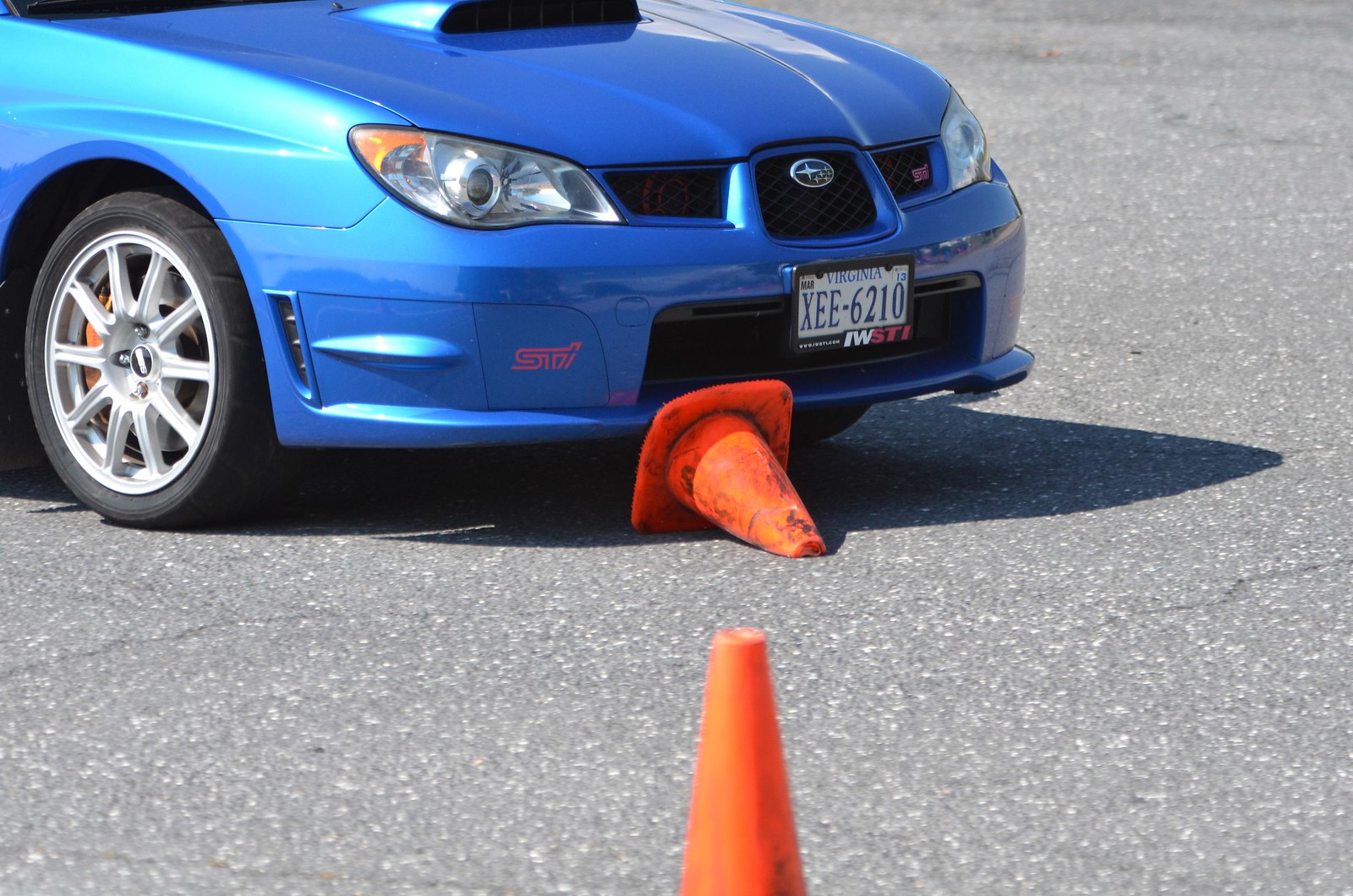This image depicts the front half of a bright blue car, identified by its Virginia license plate number XEE6210, positioned on a cracked and speckled gray pavement. The right front tire and the slanted headlights of the vehicle are visible. The car occupies the top left corner and extends about two-thirds of the way to the right and down, dominating the frame. A traffic cone is wedged underneath the front bumper, lying on its side with its tip on the ground. In the foreground stands another orange traffic cone, upright. The car features black tires with silver rims, enhancing its vivid blue color against the textured surface.